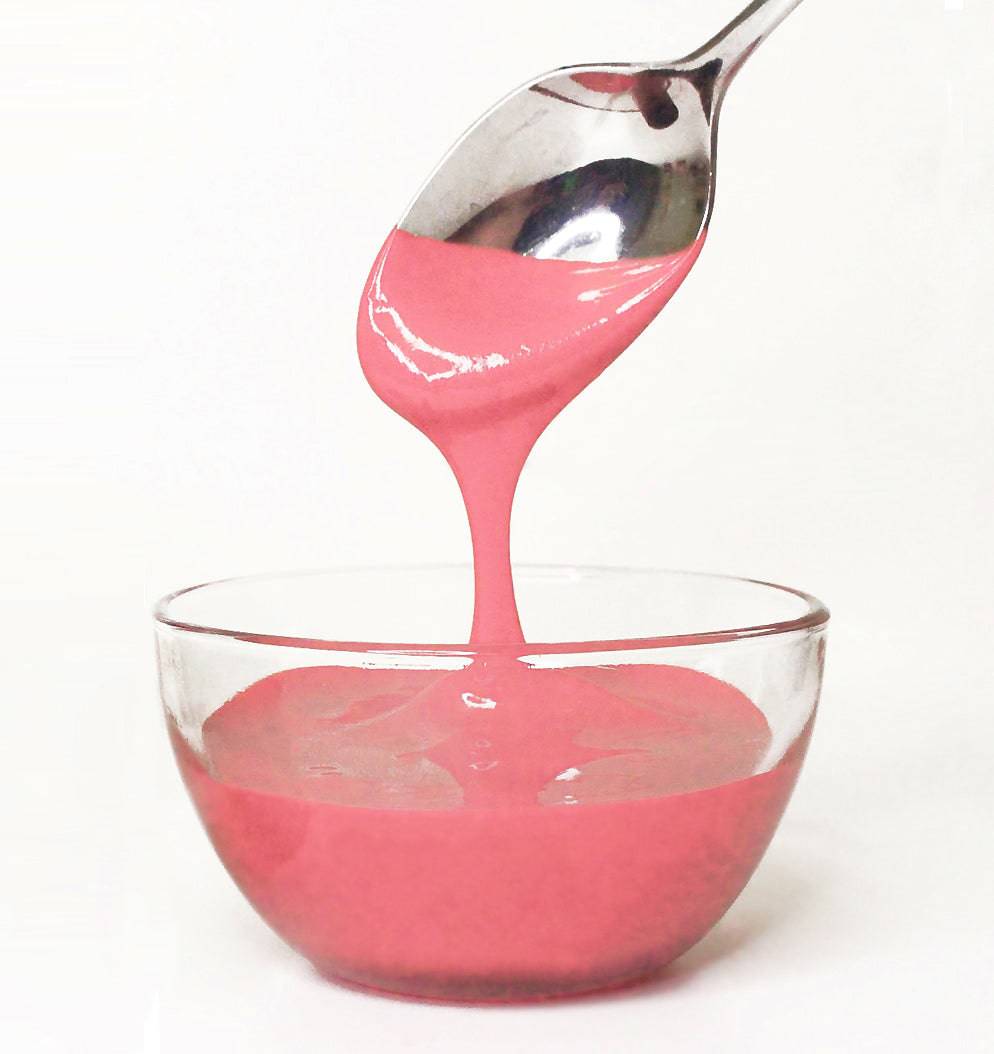In the image, a small clear bowl, made of either glass or plastic, contains a thick bubblegum pink substance. This strikingly pink liquid could be a type of dessert, possibly strawberry-flavored yogurt, pudding, or a cake batter, hinting at its vibrant color and creamy consistency. The bowl is set against a light beige or cream background, enhancing the vividness of the pink content. Resting on the bowl's edge is a shiny silver spoon, partially dipped into the pink mixture. The spoon holds some of the pink liquid, which looks poised to drip back into the bowl. The overall scene suggests a close-up and somewhat messy view of the preparation or consumption of a sweet, pink treat.